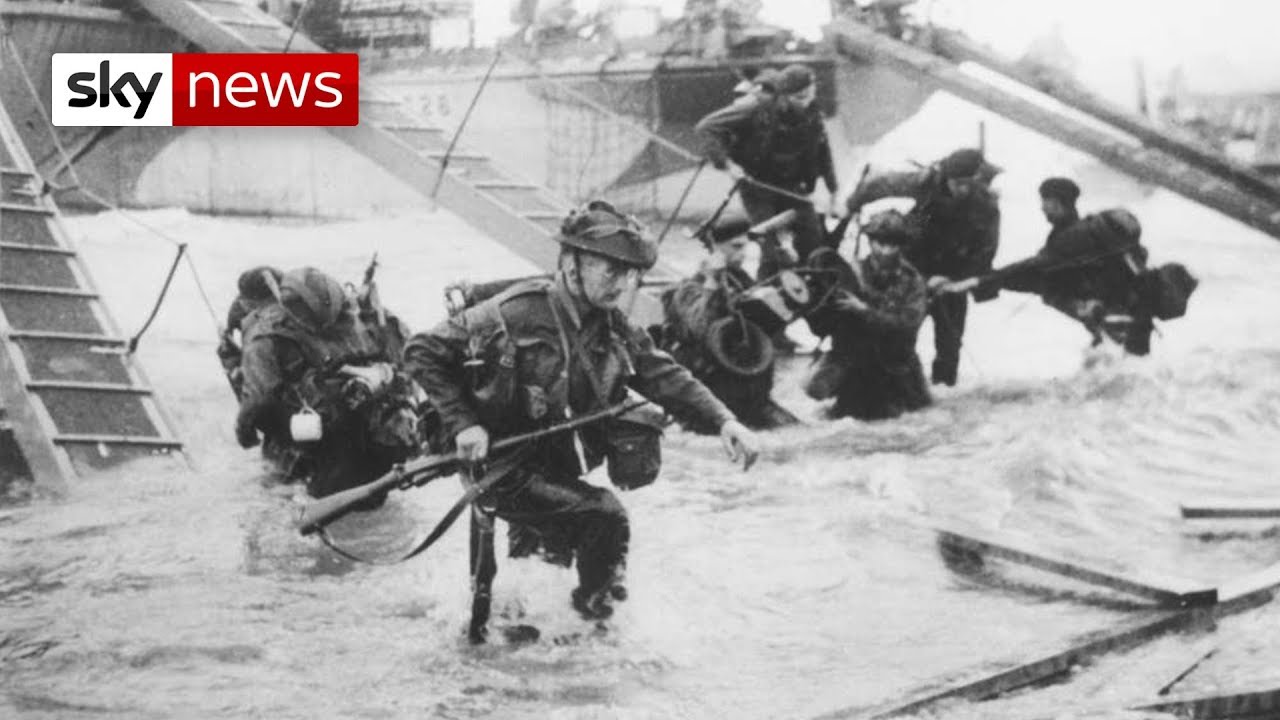This black-and-white photograph, bearing the Sky News logo in the upper left corner, captures a close-up of soldiers during what appears to be the D-Day landing in Normandy. The image prominently features water in the lower half of the frame, with soldiers wading through it, equipped with rifles and heavy gear. The soldier closest to the camera, situated center-left, wears glasses, a shallow helmet, and struggles through the water, seemingly battling both rain and the aquatic obstacle. Behind him, another soldier crouches with his face obscured. To the right, farther back, two soldiers are holding a small motorcycle, likely unloading it from a landing ship. Two more soldiers can be seen crawling down a ladder from a dark boat hull into the water, which is partially obscured by the frame. Large ladders are visible near the left of the frame, with the soldiers seemingly disembarking from these ships. Floating planks of wood in the water add to the chaotic scene as the men endeavor to bring equipment and themselves to shore, assisting each other in the process.